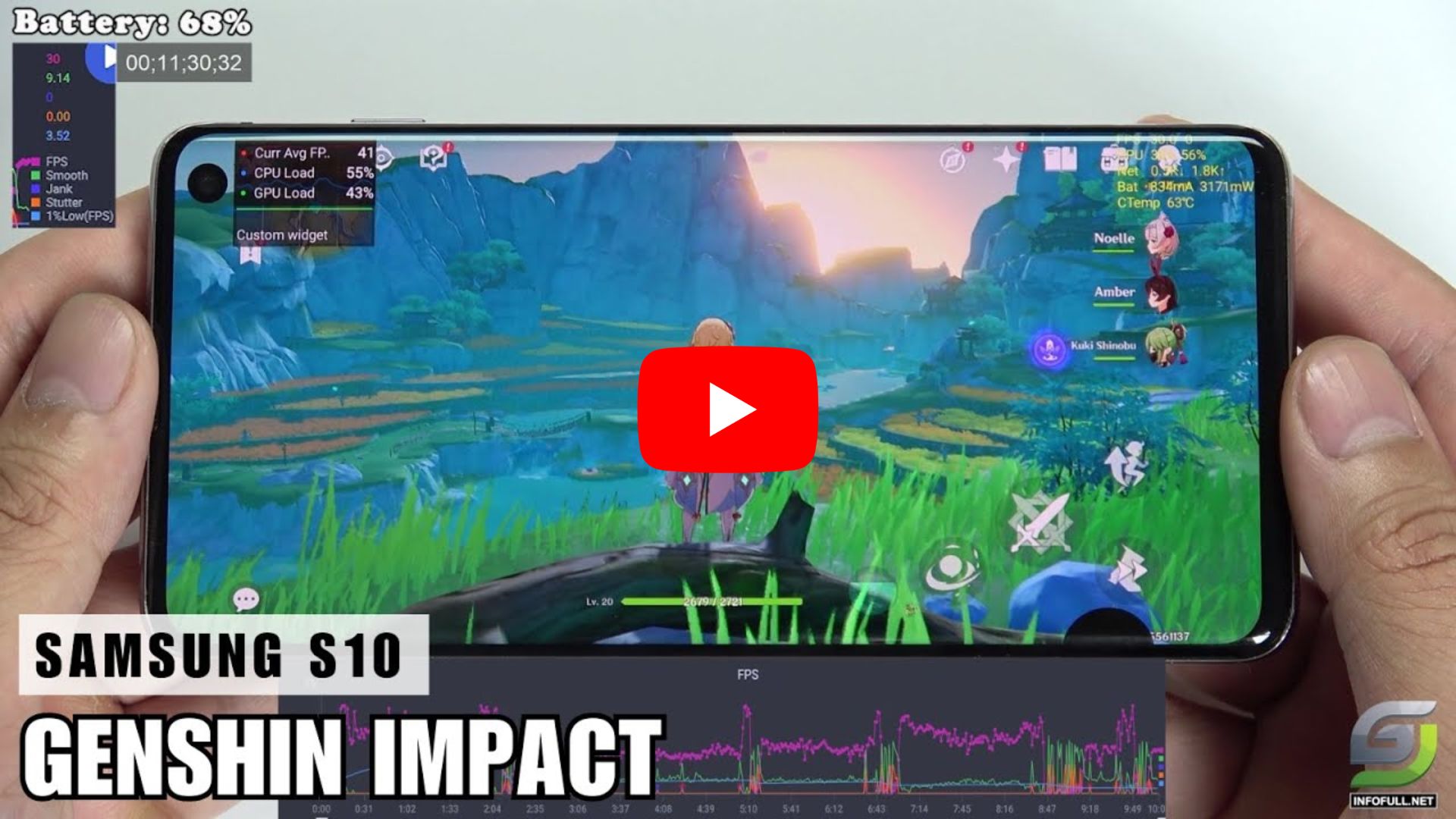The image is a detailed close-up of hands holding a Samsung S10 cell phone, displaying the mobile game Genshin Impact. The screen shows an outdoor game environment with green grass and blue mountains. The phone's interface indicates a battery level of 68%, located in the upper right corner, and the time, 11:30:32. In the bottom left corner, the text reads "Samsung S10 Genshin Impact." The bottom right corner features a logo in silver and green, which appears to be a website, though its exact URL is unreadable. This image may be a screenshot from a YouTube video, given the presence of the red YouTube logo with a white play button at the center.